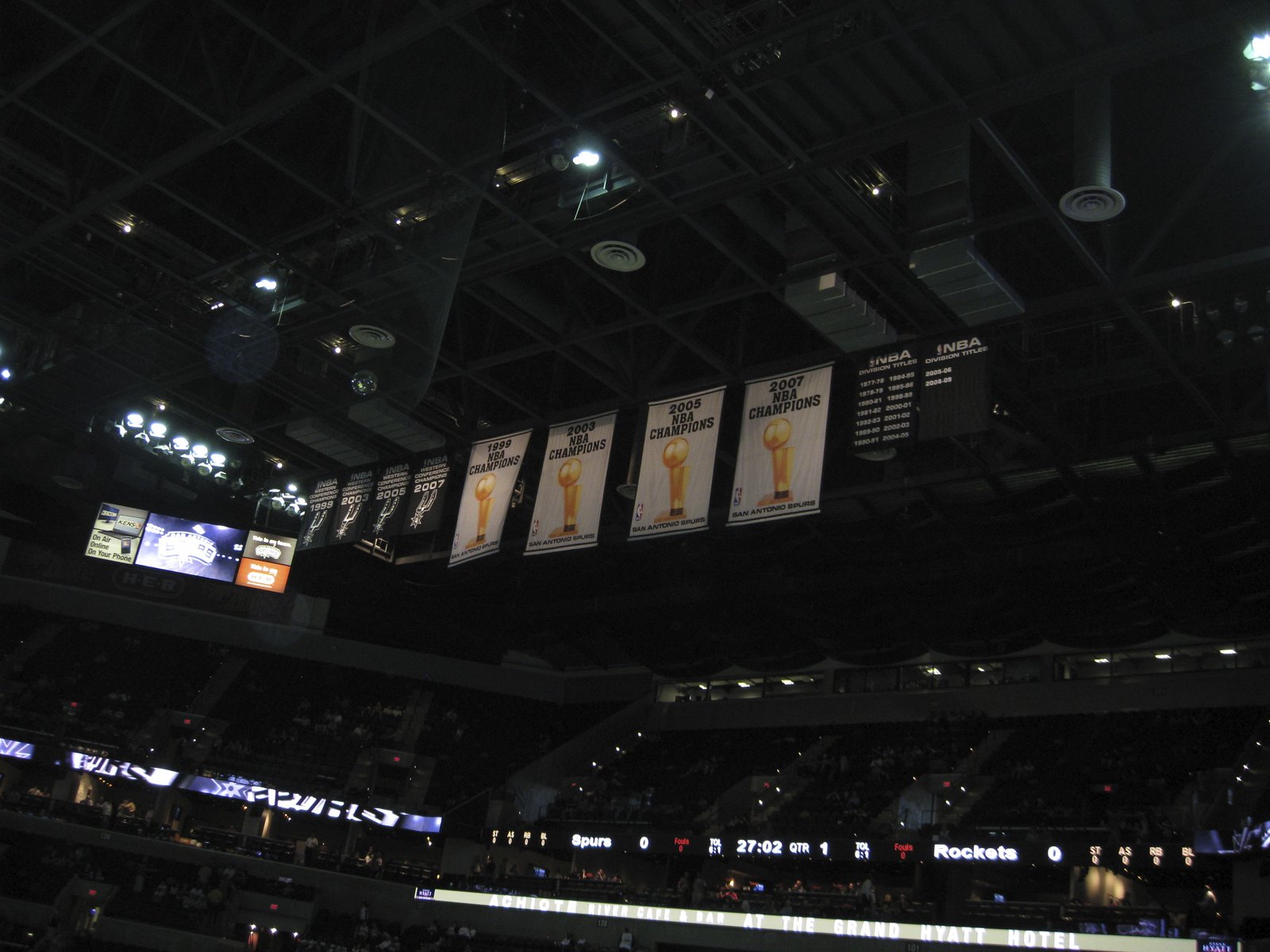The angled image captures the upper section of an arena filled with numerous NBA banners. Notably, the first four banners showcase the San Antonio Spurs logo with relevant years and white text, despite the challenging angle which makes the finer details less legible. Adjacent to these are four larger white banners, each inscribed with "NBA Champions" in black, the respective years at the top, and a trophy image. The bottom of these banners features smaller black text which remains indistinct. To the far right is a square banner, densely populated with years on the left, whereas only two years are noted on the right.

In addition, the photograph reveals structural elements of the arena, including the illuminated jumbotron and various lights affixed to the rafters. The jumbotron displays game details, including team names— Spurs and Rockets— and an ongoing time of "27:02" in the first quarter. Below, portions of the seating area are visible, with indistinct individuals seated throughout. The LED panel in the middle of the seating area shows several notations, contributing to the immersive sporting environment. Despite the overall darkness and indistinct quality, the image vividly encapsulates the celebratory spirit of the arena with its profusion of historical NBA champion banners and active game atmosphere.